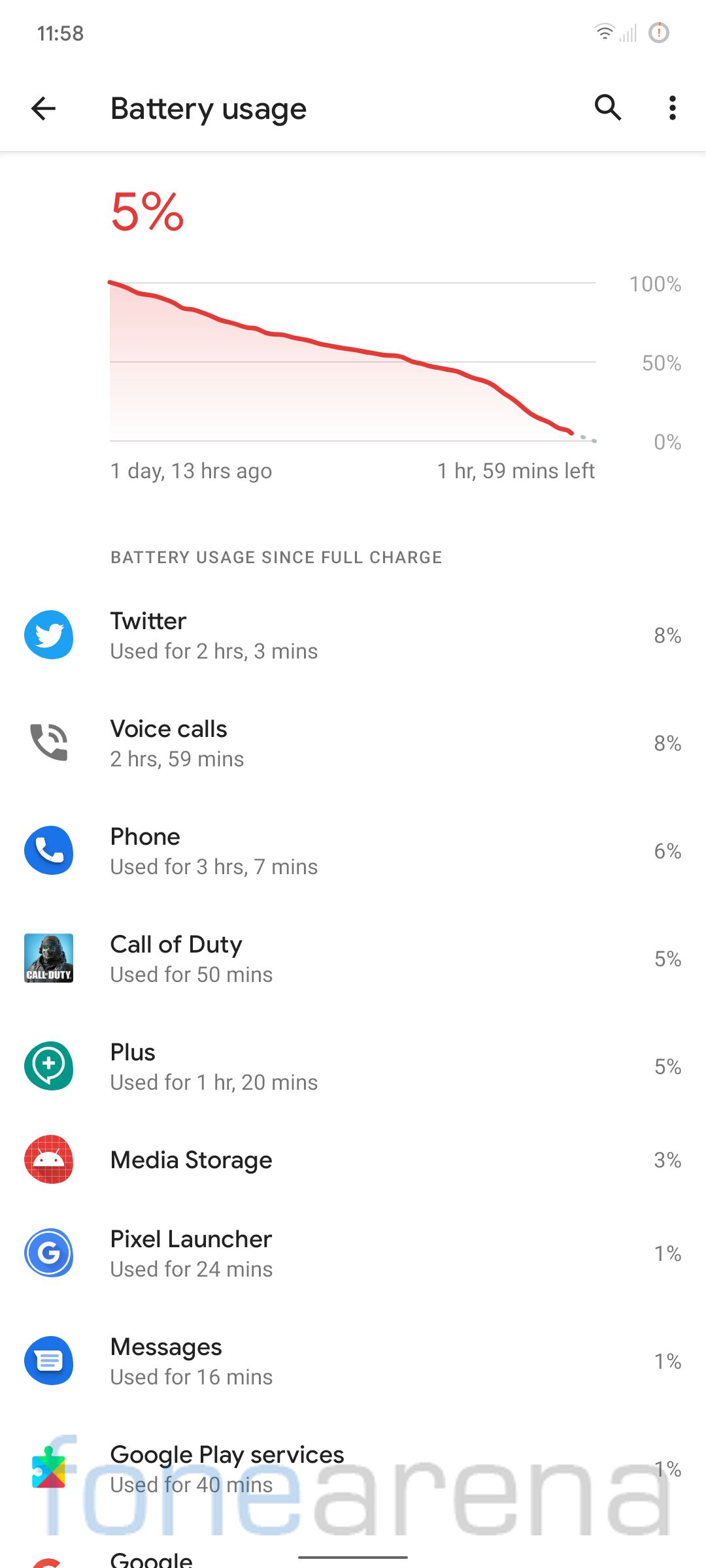The image displays a slightly blurry screenshot of a smartphone's battery usage summary. At the top, the time is noted as 11:58, with an arrow pointing left and the text "Battery Usage" beside it. Below, highlighted in red, is the current battery level at a critical 5%. A graph illustrates battery depletion from 100% to 0%, with a red line steeply descending from the top to the bottom of the chart, indicating rapid battery drain. The time since the last full charge is recorded as 1 day and 13 hours, with an estimated 1 hour and 59 minutes of battery life remaining.

Further down, under the section titled "Battery usage since full charge", is a detailed breakdown of battery consumption by various apps and system functions. The following usage statistics are listed:

- **Twitter**: 2 hours and 3 minutes, consuming 9% of the battery.
- **Voice calls**: 2 hours and 59 minutes, consuming 8%.
- **Phone**: 3 hours and 7 minutes, consuming 6%.
- **Call of Duty**: 50 minutes, consuming 5%.
- **Plus**: 1 hour and 20 minutes, consuming 5%.
- **Media storage**: Contributing to 3% of total battery usage.
- **Pixel launcher**: 24 minutes, consuming 1%.

Each app listed includes its respective icon to the left, with the percentage of battery usage clearly indicated on the right side.